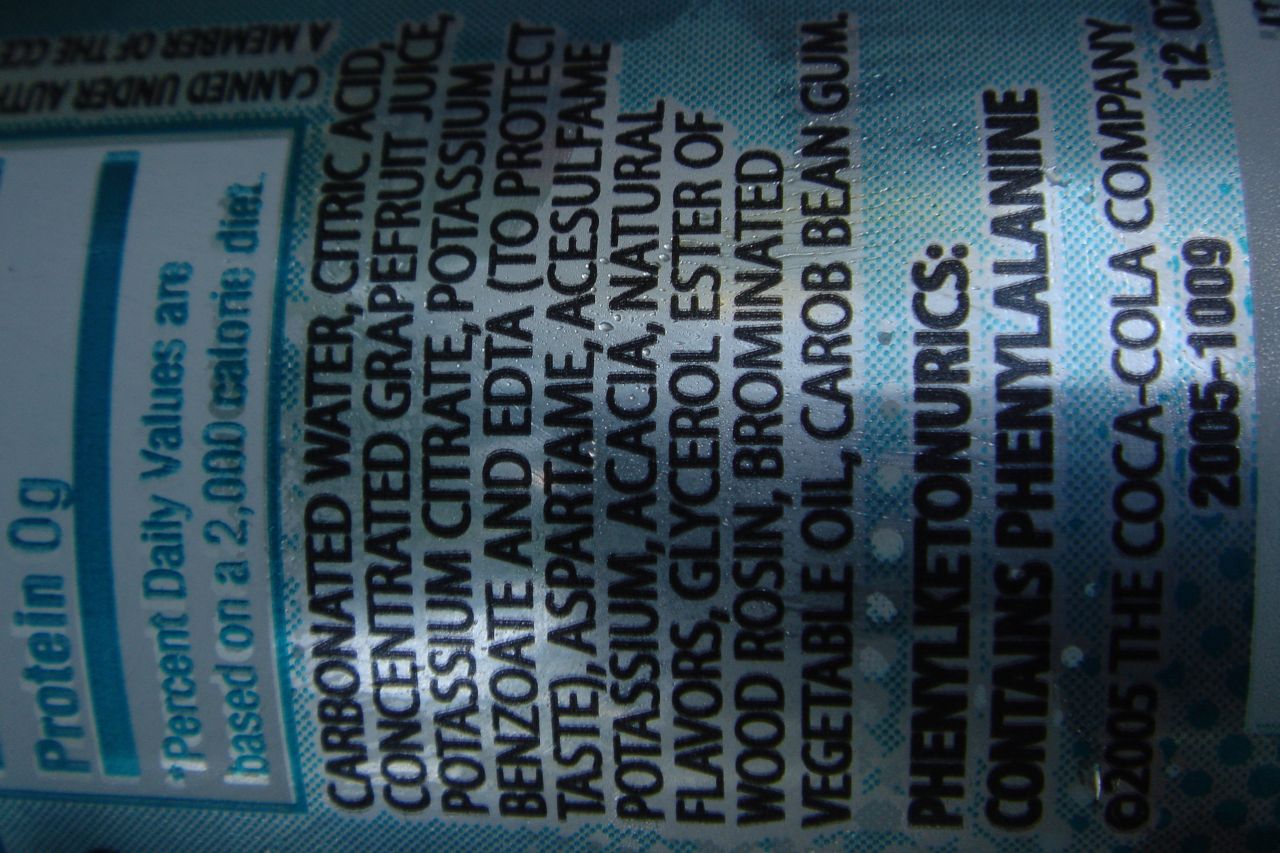The image is a sideways photograph of the ingredient label on a can of a food or beverage item, possibly a soda. The background of the can features a pattern of small blue dots. The text on the label is primarily black, with some words highlighted in blue for emphasis.

At the top of the label, it states "Protein 0g," followed by an asterisk and the note "Percent Daily Values are based on a 2000 calorie diet." The ingredient list follows: "Carbonated water, citric acid, concentrated grapefruit juice, potassium citrate, potassium benzoate (preservative), EDTA to protect taste, aspartame, acesulfame potassium, acai, natural flavors, glycerol ester of wood rosin, brominated vegetable oil, and guar gum." 

Additionally, there is a warning for individuals with phenylketonuria: "Phenylketonurics: Contains phenylalanine." The bottom of the label features a copyright notice: "© 2005 The Coca-Cola Company."